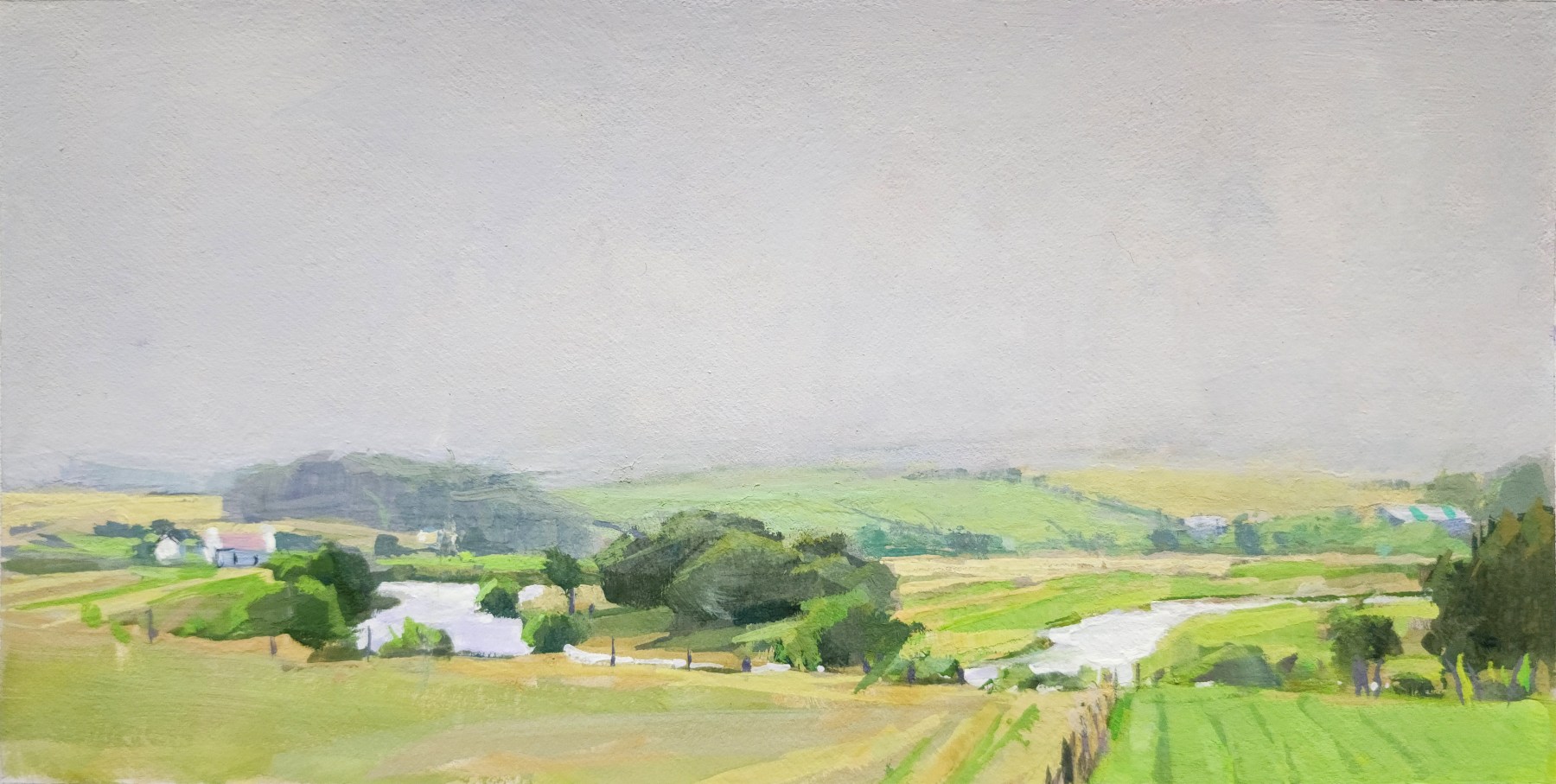This watercolor painting, viewed from an elevated vantage point, offers an expansive aerial perspective of a typical farmland scene. Dominating the scene, the sky is painted in a hazy, dark green and gray hue, suggesting an afternoon setting with no discernible sun or clouds. In the right-hand portion of the painting, lush green fields are interspersed with darker green trees, bordered by a distinct tree line that separates them from the dried-out, plowed fields on the left. A meandering creek or stream runs through the landscape from left to right, flanked by plentiful trees on both sides, suggesting an ample water supply for the farmland.

In the far left background, there is a homestead featuring a prominent white farmhouse with a red, somewhat faded roof, possibly accompanied by an additional barn-like structure set further back. On the right, the stream continues its path, bordered by trees and an extensive fence that encloses portions of the property. Further into the background, green hills and valleys seamlessly blend with orange plowed fields, enhancing the scene's depth. Despite the absence of any people, the painting vividly details the quintessential elements of a serene, working farm.